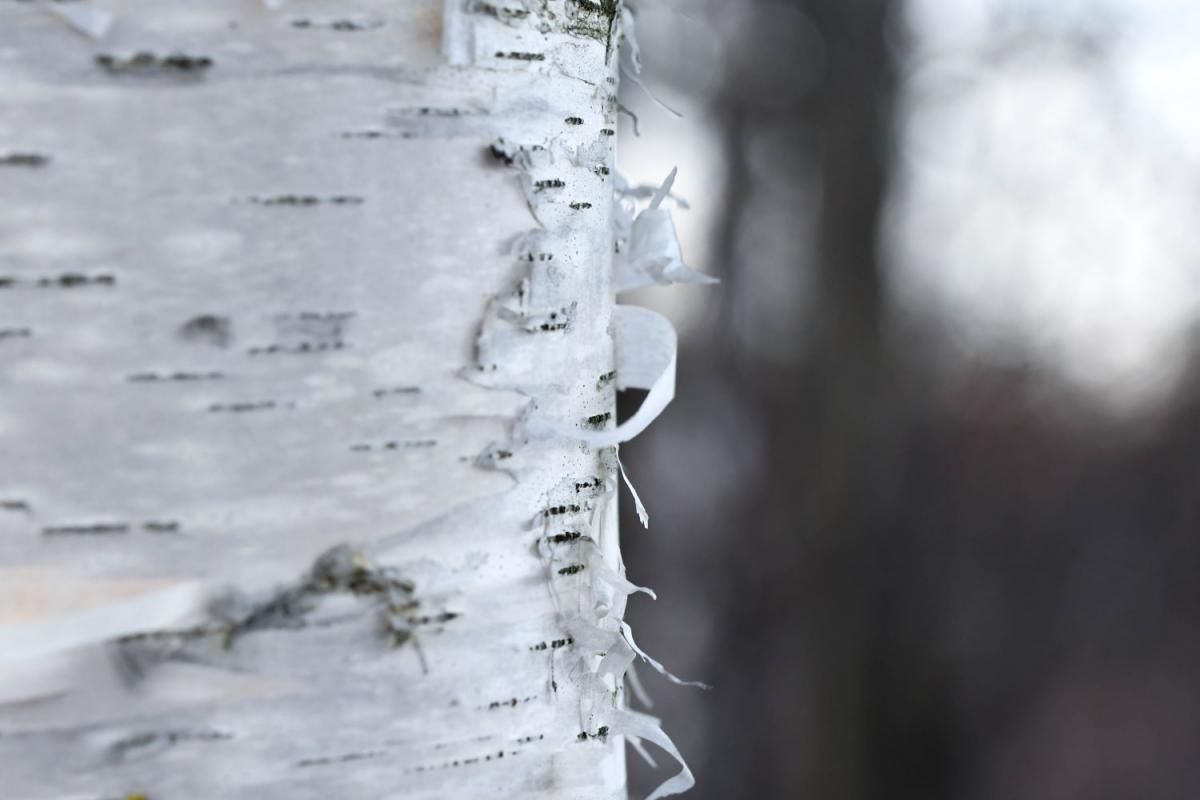This close-up daytime photograph, approximately six inches wide and three inches tall, features the detailed trunk of a birch tree dominating the left side of the image. The white bark of the tree is interspersed with small, horizontal black dots, giving it a distinct and textured appearance. Strips of the bark are peeling away, reminiscent of thin, curling shreds of tissue paper. The right side of the photograph is blurred, with hints of a wooded area in the distance. Bright white spots and a touch of blue in the upper right corner suggest sunlight filtering through the forest canopy, contrasting with a dark brown, indistinct background to the right, possibly another tree trunk out of focus. The overall color palette is a serene mix of white, gray, and subtle hints of blue, evoking a calm, natural setting.